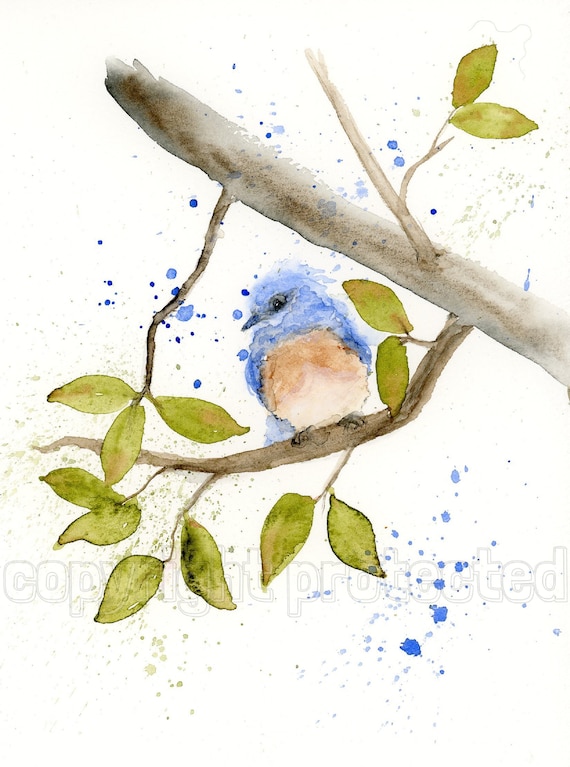This watercolor painting, set against a very light off-white background, features a prominent branch extending from the right-hand side towards the upper left. This main branch, depicted in light brown and light gray hues, supports several smaller branches and clusters of olive-colored leaves. Notable among these branches is one sweeping downwards with a delicate array of leaves. Perched gracefully on this lower branch is a small bluebird. The bird's head and back showcase vibrant blue feathers, transitioning to a lighter brown on its belly that turns whitish towards its stomach. The bird's finer details include a small blue beak, a black eye, and tiny black feet. Surrounding the bird and the branches are numerous blue paint splatters, along with a few tiny olive-colored splatters that add an artistic touch. At the bottom of the artwork, a watermark with white and gray outlines reads "Copy Protected" or "Copyright Protected."